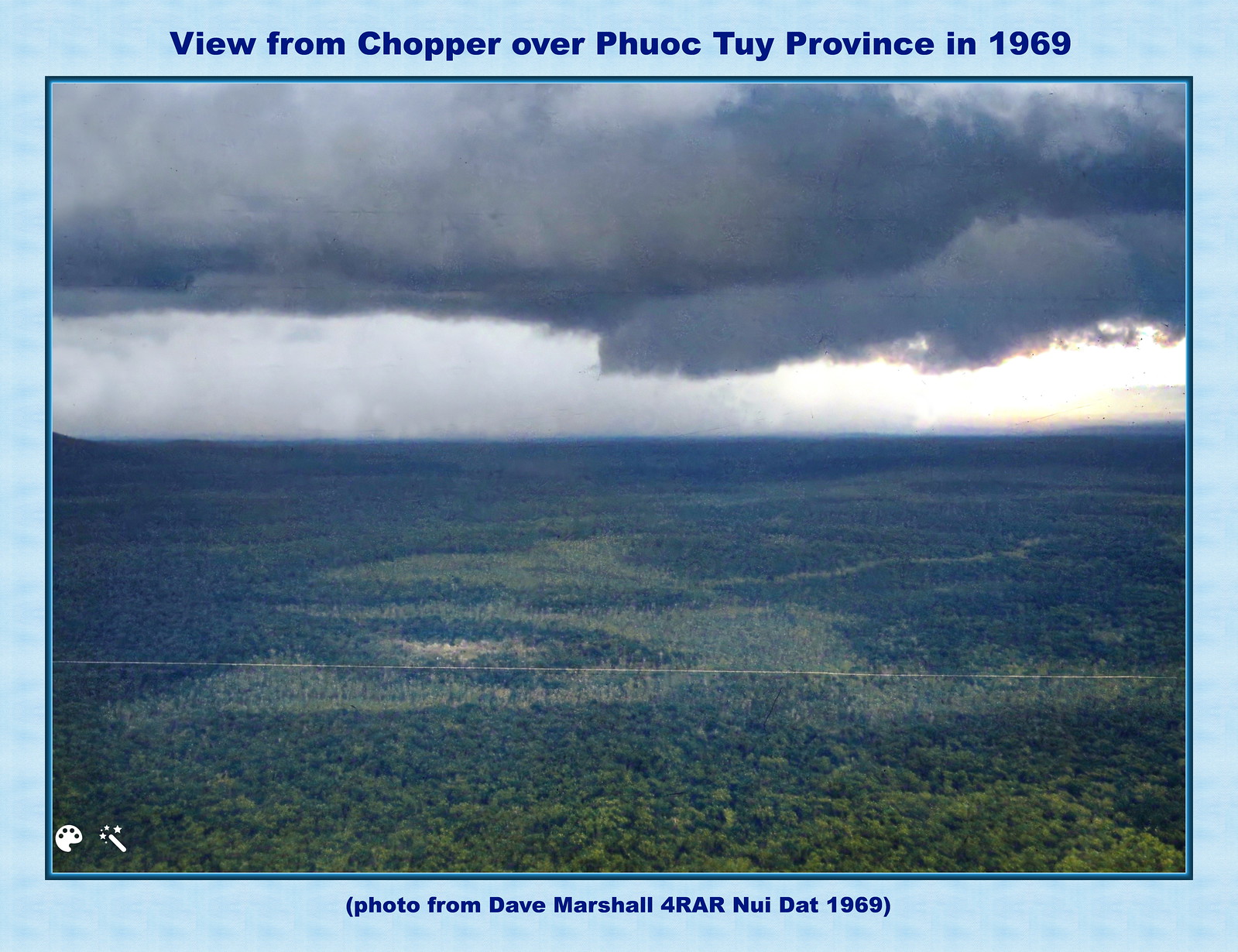The image depicted in the postcard presents an aerial view from a helicopter over Phuoc Tu Province in 1969. The photograph, taken by Dave Marshall of 4RAR and labeled as "Nui Dat 1969," captures a dense expanse of vibrant greenery beneath a moody, overcast sky. The top of the image showcases dark clouds hinting at an impending storm, with occasional breaks where sunlight peeks through. The landscape below is primarily an extensive forest with sporadic patches of lighter, possibly shorter, vegetation, creating a rich tapestry of green hues that suggest a warmer climate. Surrounding the photograph is a light blue trim, with a darker blue border encapsulating the picture part of the postcard. The text “View from Chopper over Phuoc Tu Province of 1969” is displayed prominently in dark blue on the top border. The bottom left corner of the image features small, white logos—one resembling a paint palette and the other a wand with stars, reminiscent of editing tools from a paint program. The overall aesthetic and color scheme give the postcard an aged, historical feel.